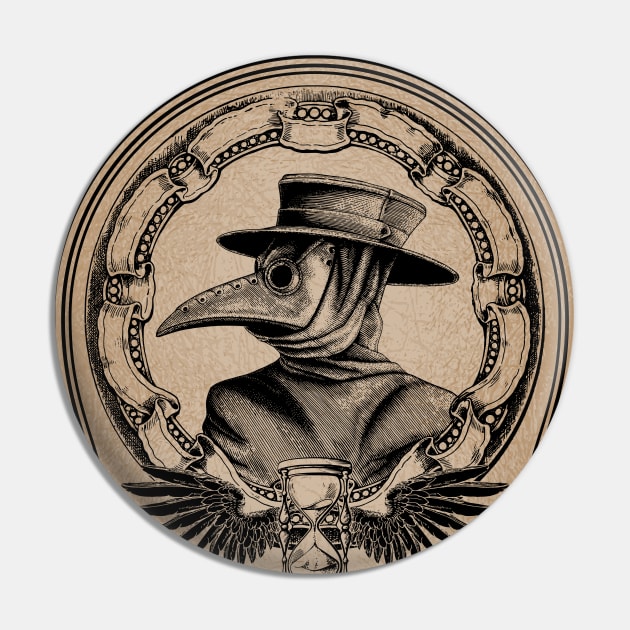This round illustration features a cartoon-style depiction of a historical "Plague Doctor" character, set against a flat gray background. The Plague Doctor, often associated with the 17th-century bubonic plague, is illustrated wearing the iconic bird-like mask and a wide-brimmed hat. The detailed costume, traditionally used by doctors to protect themselves from airborne diseases, also includes a long cloak. Encircling the character is an ornate wreath-like border. Below the Plague Doctor, there is an hourglass adorned with two wings, symbolizing the passage of time and perhaps the fleeting nature of life during plague eras.